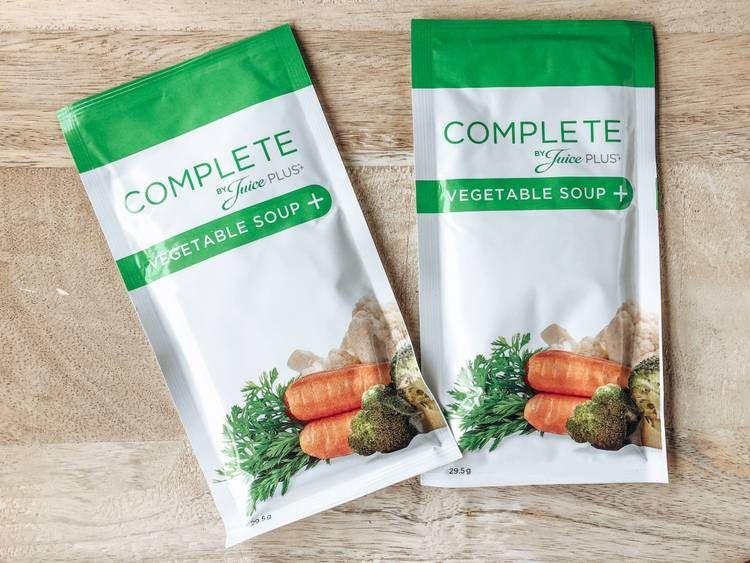This image showcases two identical packets of Complete by Juice Plus Vegetable Soup mix, positioned on a close-up, light brown wooden surface. The packets, which are taller than they are wide, are predominantly white with a clear emphasis on green detailing. Each packet features a prominent green band at the top, which reads "Complete by Juice Plus." Below that, a second green band displays the text "Vegetable Soup" in white font, followed by a plus symbol. Near the bottom of the packets is a photographic depiction of various vegetables, including carrots with visible green tops, broccoli, cauliflower, and possibly some cabbage. Each packet weighs 29.5 grams. One packet is oriented straight up, while the other is slightly tilted to the left.